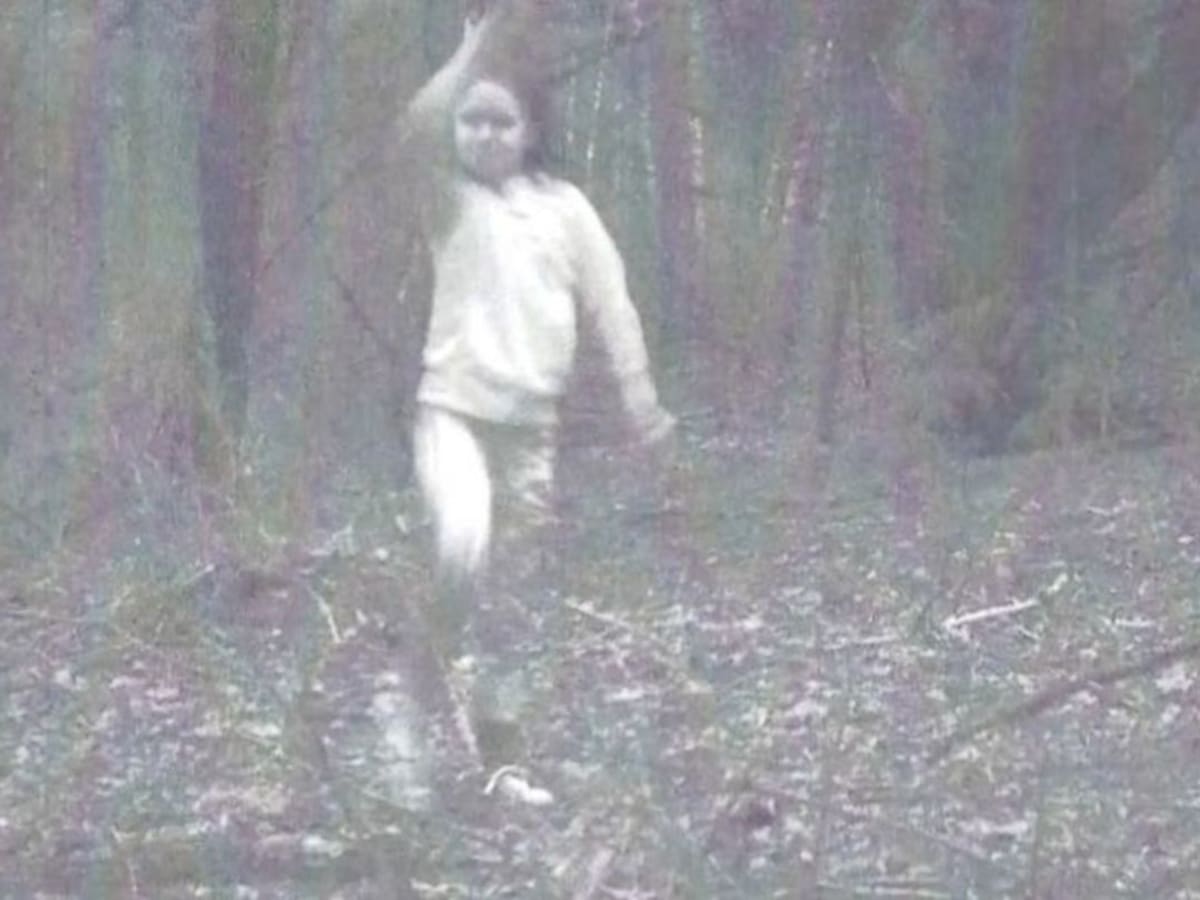The image is an old, black-and-white photograph, possibly from around the year 2000, though it might be much older or just poorly preserved. The photograph is quite blurry, suggesting it may be a copy of an original photo, perhaps even printed on plain paper.

In the image, there is a child who appears to be a girl, although it's somewhat difficult to determine the child's gender with certainty. She is wearing a white long-sleeve top and white pants, which appear dirty and muddied, blending with the background to some extent. The child is also wearing what seem to be white tennis shoes. She stands outside in a forested area, surrounded by leaf litter, dirt, sticks, and possibly patches of grass. Behind her, there are trees that might be pine trees, given the apparent lack of visible leaves on them.

The girl is in a bit of a clearing, with one arm raised slightly and the other down by her side, possibly in motion as her right knee is bent. She is looking directly at the camera, but her face is blurry and lacks clear detail. The overall scene gives a sense of an older time captured in a moment within a natural, wooded environment.